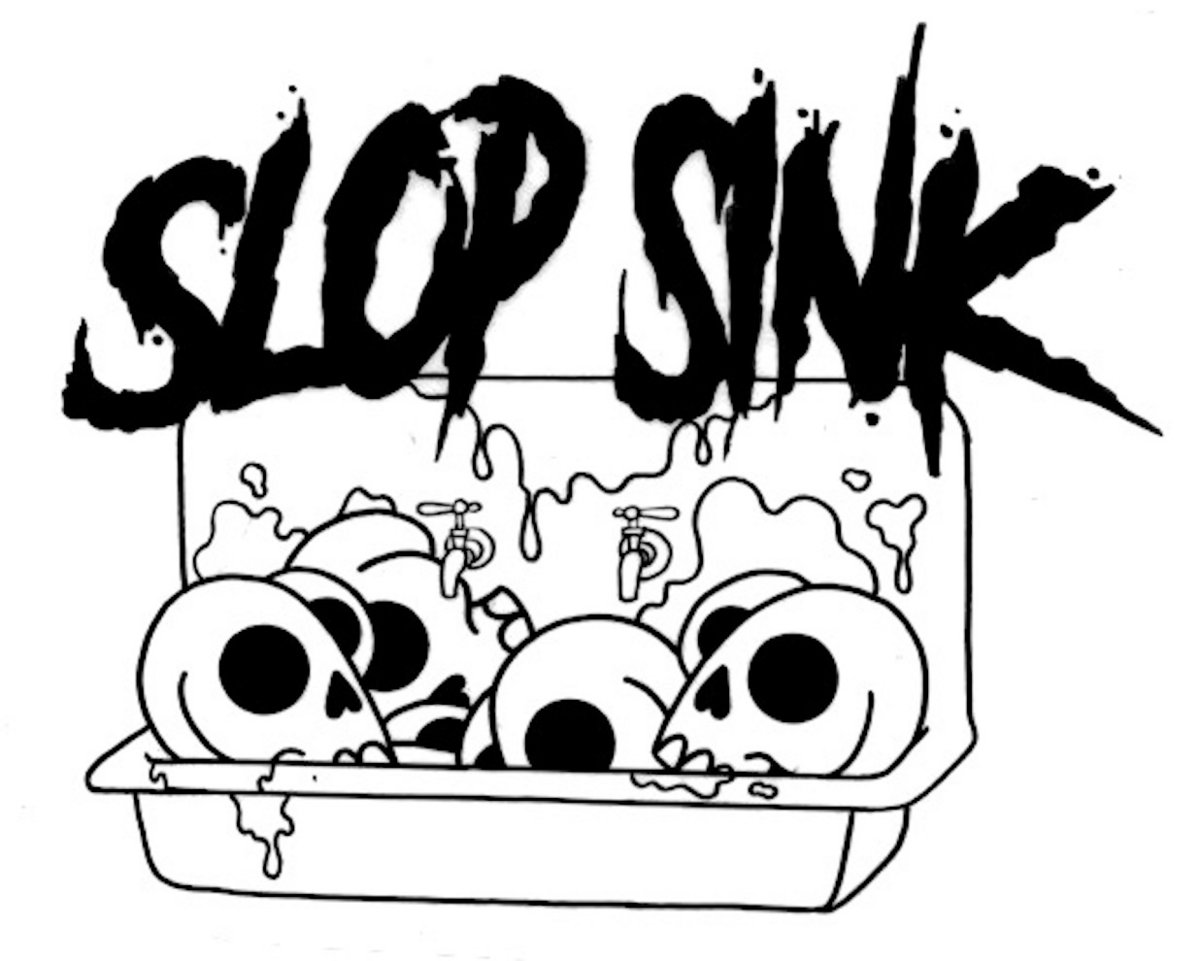The image features a black and white drawing devoid of any color, evoking the simplicity of a coloring book page, potentially suited for an adult coloring book due to its eerie content. Set against a solid white background, the central focus is a large, trough-like porcelain sink positioned towards the bottom of the image. The sink is detailed with a high vertical back and two faucets, implying an industrial design.

Within the sink, a chaotic arrangement of about half a dozen white skulls is depicted, their macabre appearance emphasized by big, circular eye sockets and inverted heart-shaped nose holes. These skulls are randomly oriented, facing various directions, further adding to the disordered motif. Surrounding the skulls, in and around the sink, is a noticeable mess suggestive of splashes of water, enhancing the chaotic scene.

Above this unsettling scene, the words "Slop Sink" are prominently displayed in large, messy capital letters, appearing as though they are dripping, perhaps mimicking blood or paint. This text anchors the image composition from the top, its sinister font contributing to the overall eerie atmosphere. The entire illustration, characterized by its stark black outlines against a white backdrop, strikes a haunting yet intriguing visual balance.